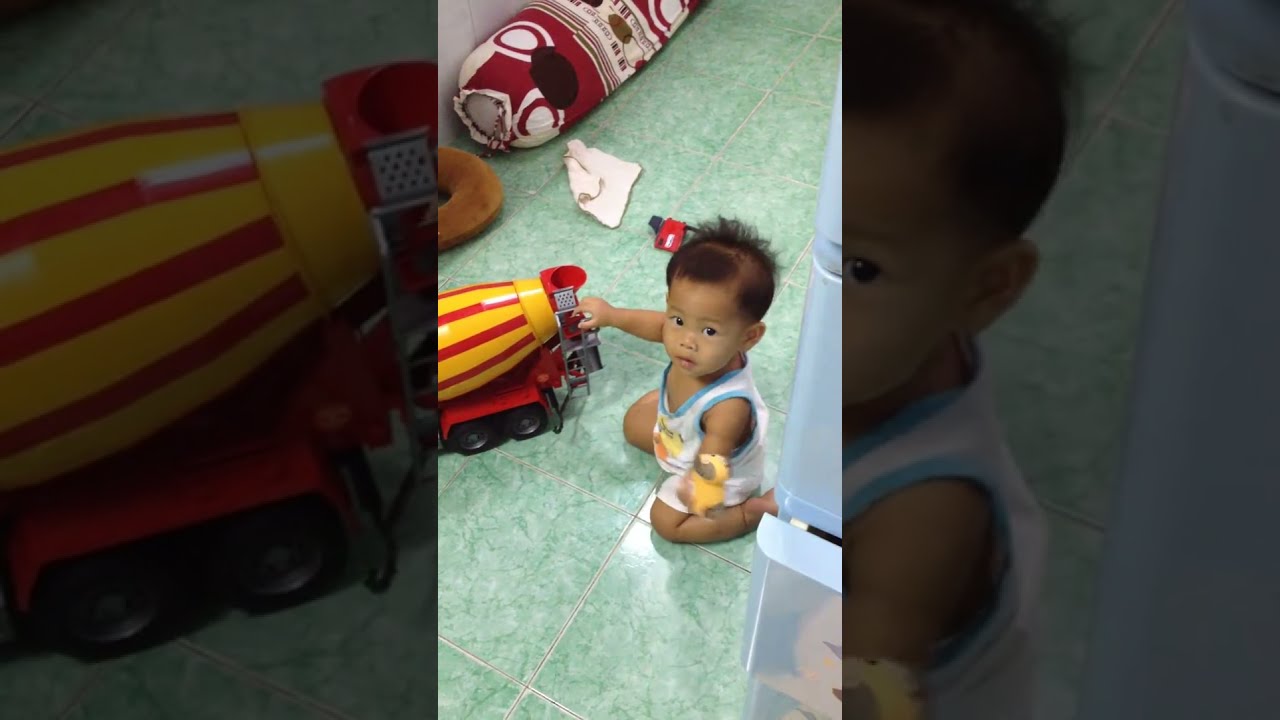A young toddler with dark brown skin, approximately one to two years old, is kneeling on a green marble tiled floor. The toddler is dressed in a white tank top with blue edging and is bare-legged, wearing only short pants. In their right hand, they appear to be holding a white diaper or piece of cloth. The toddler's attention is fixed on a colorful toy truck, designed to resemble a cement mixer, which is predominantly red with yellow and orange highlights. The cylindrical mixing drum of the truck features distinctive red striping. Next to the truck on the floor is a brown, circular, pillow-shaped toy, accompanied by another red and white item. The image is framed by vertical black rectangles on either side, focusing on the central subject—the toddler and the vibrant toy truck. The scene suggests a commercial setting rather than a home environment.